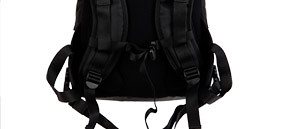The image depicts a medium-sized, rectangular black backpack viewed from the back. The background is white, which contrasts with the black color of the bag. The backpack features multiple straps, including shoulder straps with adjustable buckles for fitting adjustments. Visible at the bottom are the ends of these shoulder straps with the adjustable mechanisms and additional straps for further adjustments. There is a zipper on the right side near the bottom part of the bag. Although it’s hard to discern specific details, there's no text present on the backpack. The lighting and angle make it challenging to see the full depth and dimensions of the bag.